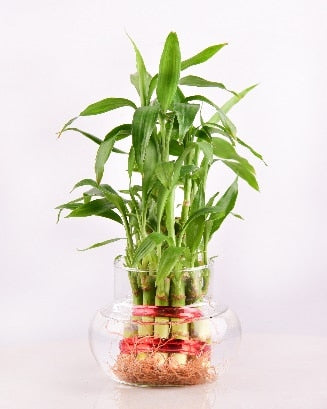This photograph depicts a bamboo plant arrangement inside a clear, short glass vase with a wider, rounded bottom half-filled with clear water. The bamboo stalks, featuring green rod-like stems, extend upwards, showcasing long, narrow green leaves that are pointed at the ends. The bases of the bamboo stalks are tied together with two red ribbons or straps, and at the very bottom of the plant, thin pink roots are visible, tangled together. Some light yellow plant material, possibly moss or another plant, is present around the roots. The entire arrangement is situated on a white surface with a pure white background, enhancing the vibrant greenery of the bamboo.